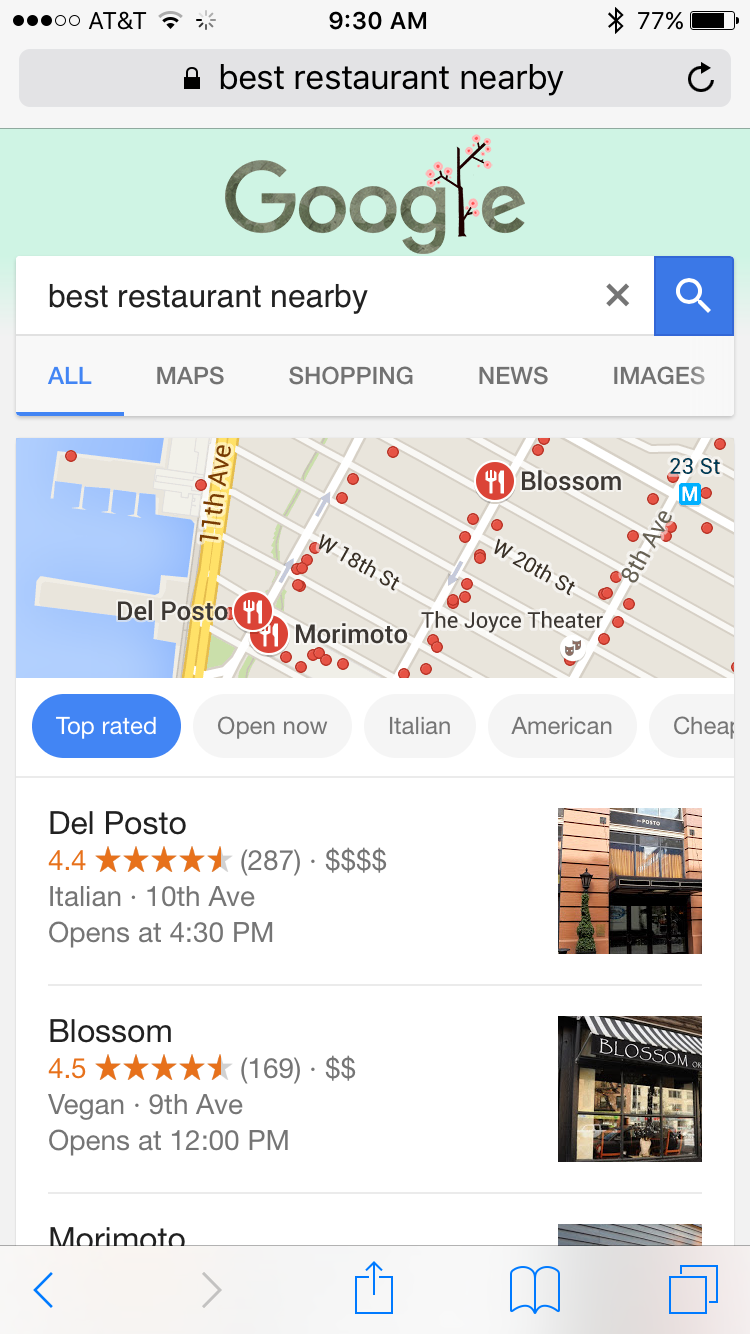A detailed screen capture of a smartphone displaying a search for nearby restaurants. At the top left, there are three solid black dots followed by two clear ones. To the right, it indicates "AT&T" with a Wi-Fi signal icon and a sunshine symbol. Centered at the top in bold black text is the time "9:30 AM." On the upper right corner, there's a Bluetooth icon, a battery level at 77%, and a black battery icon.

Beneath that, a mid-tone gray bar features a lock symbol, the text "Best Restaurant Nearby" in black, and a reload button on the right. Directly below, a mint green banner displays "Google," where the "L" is styled as a cherry blossom tree. There's a white search bar underneath with the text "Best restaurant nearby," and a blue square with a magnifying glass icon on the right.

The menu options below include "All," "Map," "Shopping," "News," and "Images." A rectangular street map section follows, marked with red icons featuring a white knife and fork indicating restaurant locations. The "Top Rated" filter is selected in blue, with a list of top-rated restaurants below:

1. **Del Posto**: Rated 4.5 stars with an icon on the right showing an exterior view of the building.
2. **Blossom**: Rated 4.5 stars with an image on the right displaying a black awning that reads "Blossom" in white text.
3. **Morimoto**: Only partially visible, showing the name "Morimoto" and the top of an associated image icon.

At the very bottom, a gray bar hosts navigation icons: a blue left arrow, a gray right arrow, a blue square with an upward arrow, an open book in blue, and two overlapping squares outlined in blue.